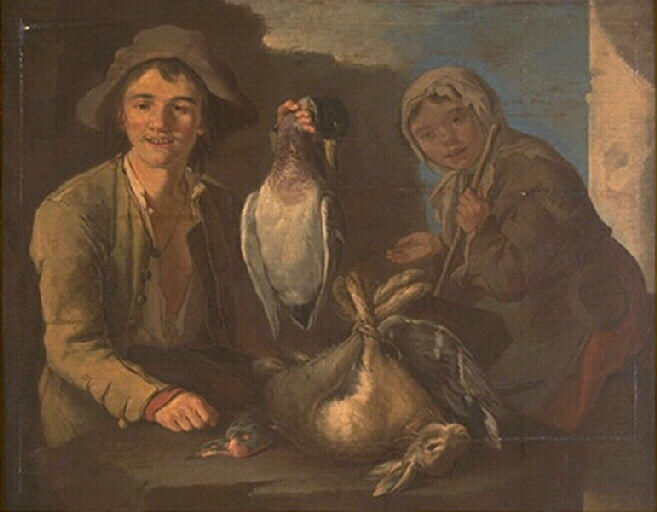This detailed painting depicts a scene likely set in historic times, showcasing a teenage boy and a young woman in modest, worker's attire indicative of a rural or medieval period. The boy stands on the left, slightly smiling as he holds a freshly hunted duck by its neck with his left hand. He wears a fisherman's hat, a gray-brown jacket over a white shirt, and his overall appearance suggests a life of labor or hunting. 

To his right, the young woman also appears in worker's clothes, including a bonnet and a jacket, and she holds a cane or tool in her hand while gazing at the table before them. On the wooden table lies the day’s catch: a rabbit with its legs tied together and several birds, including a small blue and pink bird and a black bird, all laid out as if prepared for inspection or sale. 

In the background, the painting subtly hints at a town setting with blurred buildings and an open sky visible in the upper right corner. The expressions of the figures and the bounty on the table convey a sense of satisfaction, suggesting a successful hunt and the promise of a meal or trade.